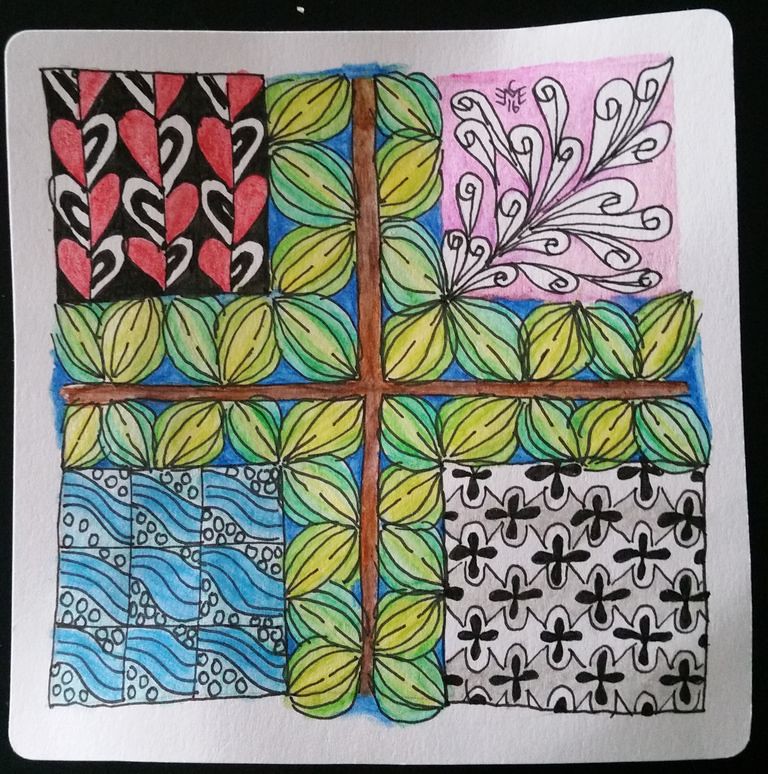This image showcases a detailed and vibrant artwork that appears to be a drawing or painting, divided into four distinct quadrants by a prominent, thin brown cross that runs from top to bottom and left to right, effectively squaring the canvas. The cross is surrounded by greenish and light yellow flower bulb-like shapes that add a decorative touch around the central cross. Each of the four quadrants has its own unique design. In the top left, red, black, and white hearts sit against a green background formed by oblong shapes converging at a point. The top right quadrant features a pink tree with paper-like leaves, growing diagonally. The bottom right quadrant is marked by black crosses with white outlines set against a checkerboard background. Finally, the bottom left quadrant contains squares resembling waves with a blue and bubbly pattern. The entire composition is framed by a black outline and a white trim, and the artwork itself rests on a black surface, possibly indicating it is part of a sketchbook page.